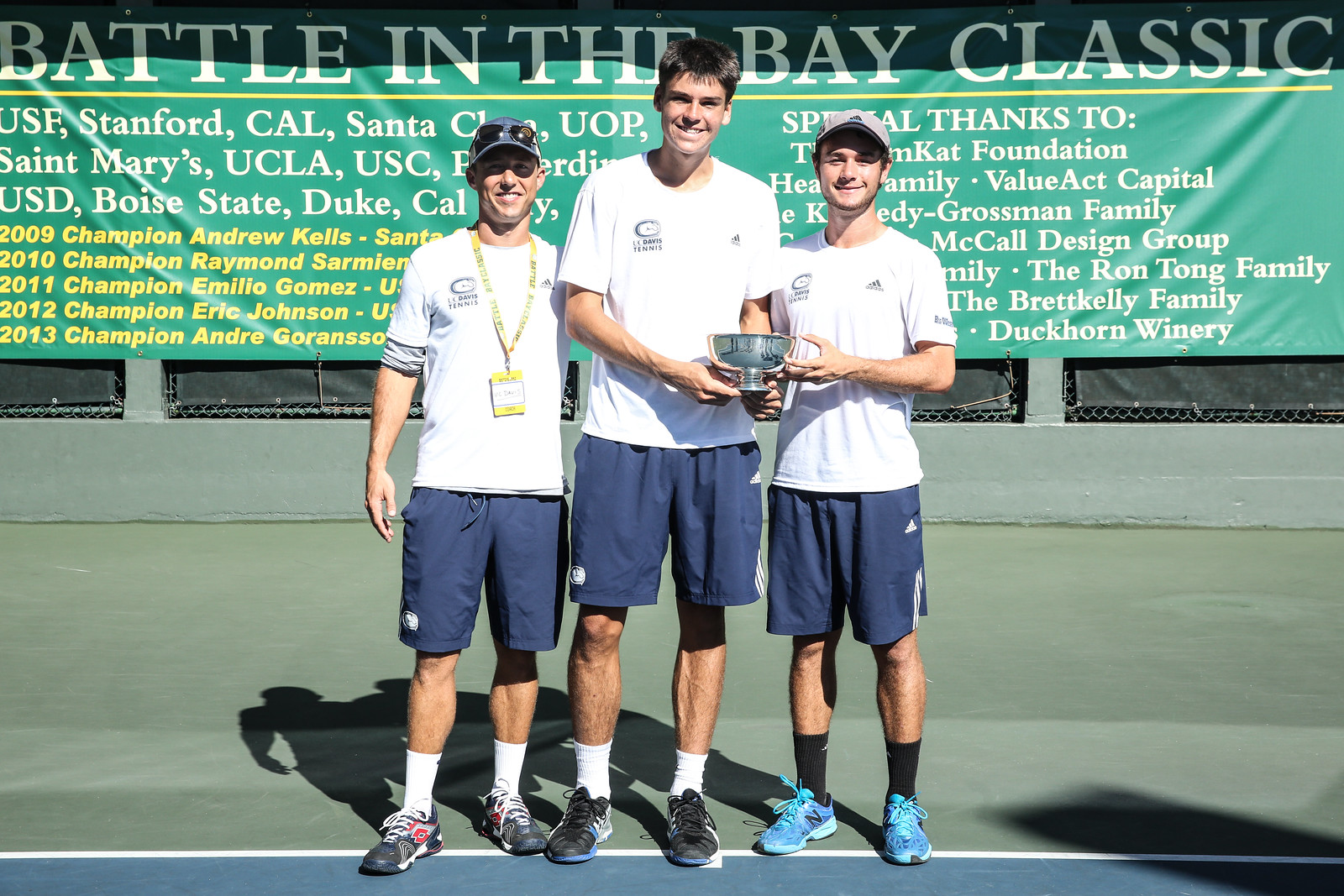In this image, three men are standing on a green and blue tennis court in front of a large green banner that reads "Battle in the Bay Classic" in prominent white font. The banner also includes acknowledgments to various foundations, families, groups, a winery, and lists champions from 2009 to 2013. The men are dressed uniformly in white short-sleeved shirts with a "C" on the chest, paired with blue shorts and sneakers—two with white socks and one with black socks. The sneakers vary in color, including gray and red, black and blue, and mostly blue with a hint of purple. The tallest of the three stands in the center, holding a silver winner's cup, while the other two men, positioned on either side, also hold similar metal vases or trophies. The men on the ends are both wearing hats; the left one sports a blue hat with sunglasses, and the right one a gray hat. The photo is taken during the day with sunlight illuminating the scene. The court has a green outer area and a blue inner area.